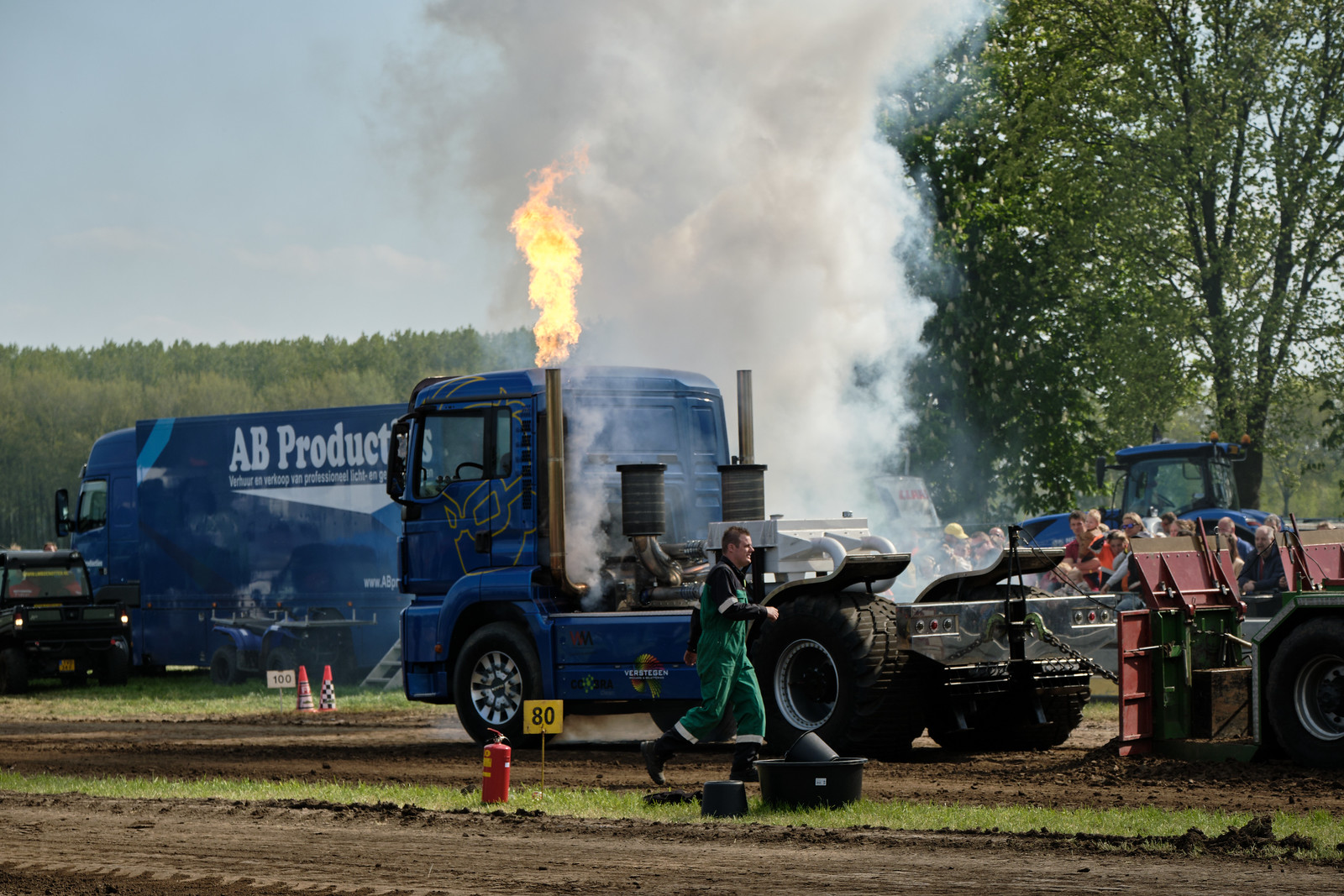In the image, set in an outdoor, muddy grassy field under a partly cloudy sky, a central blue cab-over semi-truck, marked with "AB Productions" and additional foo-writing below it, is depicted in a state of intense activity. This truck, which is positioned directly in the center, has flames erupting from one of its tall exhaust stacks and a large puff of white smoke billowing upwards. In front of the truck, there are safety cones, a fire extinguisher, and a sign marked with the number 80. A man in green coveralls, possibly a mechanic, is seen running past the truck. To the left, a wooded area is visible, contrasting with a singular large tree to the right. A crowd of onlookers, including a man holding a baby, watches the spectacle, while a group of workers, likely construction or safety personnel in matching outfits and hard hats, stands nearby. The scene appears to be set at a tractor pull event, with additional heavy machinery and tractors visible in the background, further emphasizing the rugged and dynamic atmosphere of the setting.